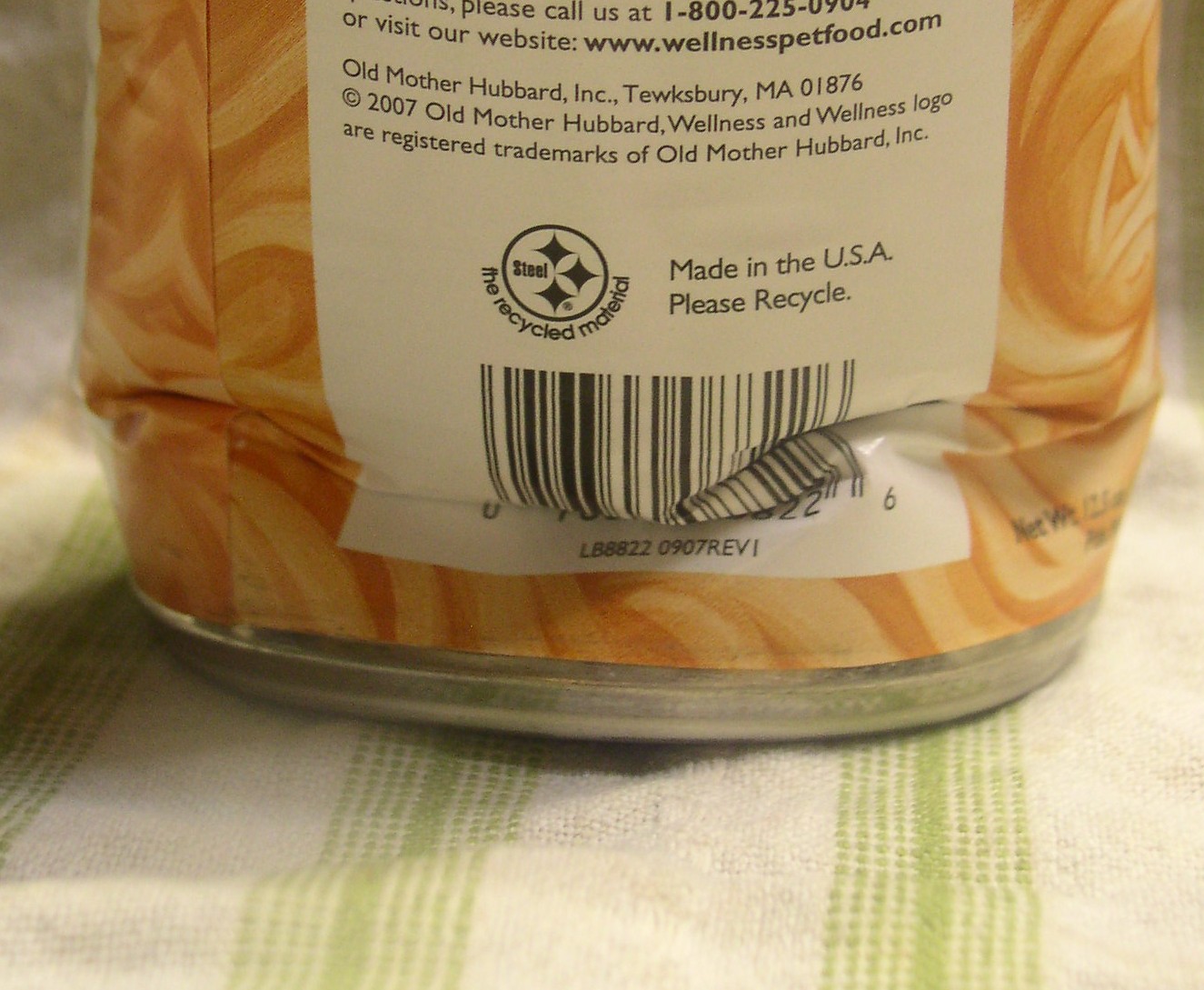This detailed color photograph captures a close-up view of the bottom of a can, which rests on a dish rag or towel. The can, which is orange with a swirly design and a metallic bottom, appears to have been damaged, resulting in a noticeable crush towards its label. The back label of the can is visible in the image; it's predominantly white, featuring a UPC symbol and a recycle symbol above it. At the top section of the label, the text reads "Old Mother Hubbard, Tewksbury Mass," followed by additional smaller text. The crushed portion of the can creates a slight shadow to the left on the towel beneath it. The towel itself is white with green accents, and the entire scene exhibits a yellowish tint, suggesting that the photo was taken under artificial lighting.